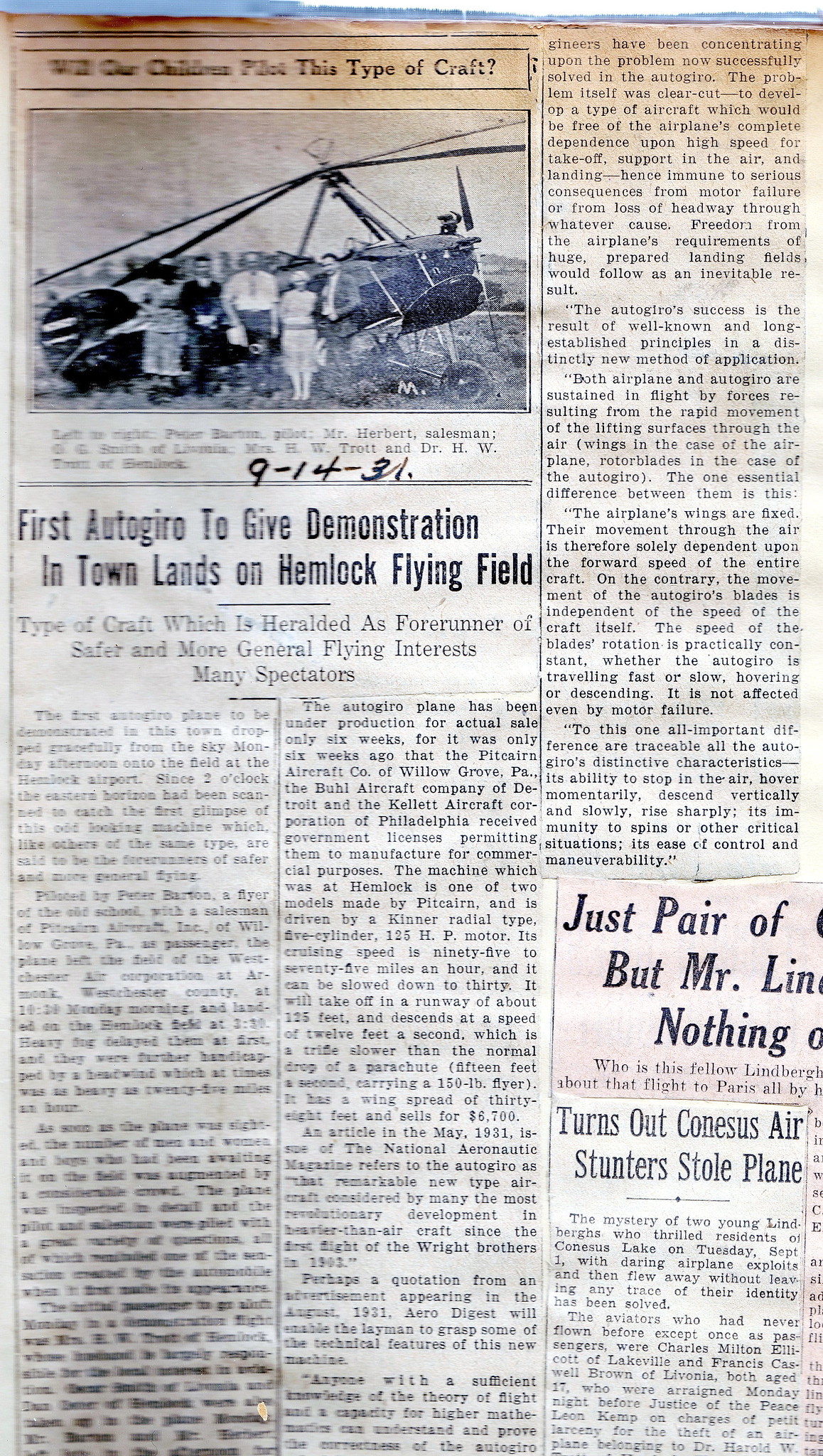The image depicts an old and weathered black-and-white newspaper clipping, arranged vertically and roughly twice as tall as it is wide. The page is divided into three horizontal sections of text, separated by lines, with a noticeable level of browning at the top, likely due to aging or sun exposure. In the top left corner, there is a black-and-white photograph of five individuals posing in front of an aircraft that looks like a hybrid between an airplane and a helicopter. This unusual craft is closely related to the newspaper headline, which reads: "First Auto Giro to Give Demonstration in Town Lands on Hemlock Flying Field." The subtitle describes the Auto Giro as "a type of craft heralded as the forerunner of safer and more general flying interests, with many spectators" present at the event. Below this, there are two more stories with headings that are partially legible, including "Turns Out Connoisseurs Air Stunters Stole Plane." Additional text is present on the right-hand side of the page and continues below. Despite some blurring, the newspaper clipping maintains clear focus on the historic significance of the Auto Giro's demonstration.